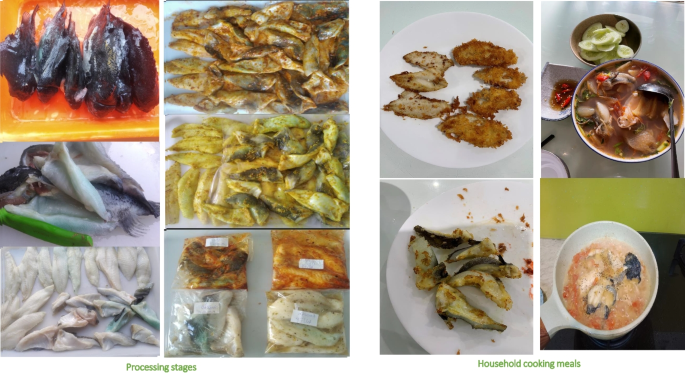The image is a highly detailed informational display depicting various stages of seafood preparation and cooking. It is divided into two distinct sections. The left section, labeled "Processing Stages" in small green text, consists of four images showcasing the transformation of what appears to be squid. The sequence begins with raw squid in an orange tray, followed by stages of cutting, seasoning, and finally marinating the pieces in plastic bags. The right section, labeled "Household Cooking Meals" in similar green text, contains four images displaying the finished seafood dishes. These include fried filets or calamari, a bowl of soup, another type of fried dish, and possibly a sushi bowl or a goulash type of seafood meal. Each section effectively illustrates the journey from raw seafood to a variety of cooked meals.